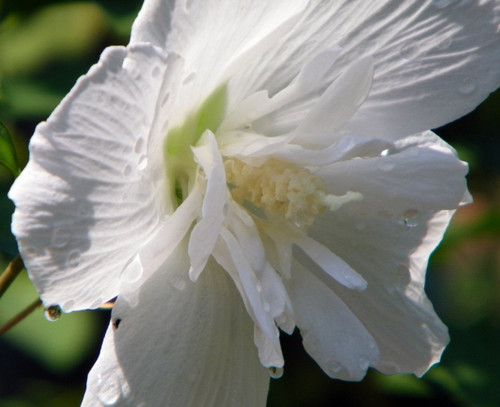The image displays a macro-scale photograph of a single, delicate white flower in full bloom, occupying most of the square frame. The background reveals blurry green leaves at the top left, bottom left, and bottom right, along with a few stems on the left side. The flower, potentially a daffodil, showcases large, slightly wrinkly white petals adorned with clear water droplets. The petals radiate outward from an off-white, textured center with hints of yellow and tiny whitish filaments. Altogether, it creates a striking and intricate visual against the contrasting green foliage. There is no text on the image.